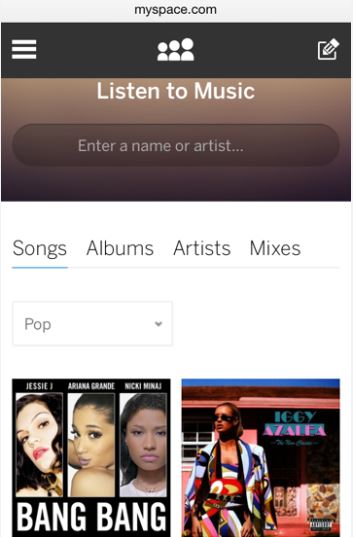The image showcases a cell phone screen displaying the MySpace.com interface. The screen has a vertical orientation, making it taller than it is wide. 

At the top, there is a thin gray band featuring the MySpace.com logo in black letters. Below this, a black panel spans the width of the screen. On the left side of this black panel, three horizontal white bars are displayed. In the center, there are three graduated images of people, represented by white circles atop semicircles. On the right side of the black panel, a white outlined square with a pencil icon is visible.

Directly beneath the black panel, a light brown section appears with the text "Listen to Music" in white letters. This transitions to a medium brown search field containing the placeholder text "Enter a Name or Artist," also in white. The panel further darkens towards the bottom before the screen transitions to a white background.

Within this white section, four options are listed in black letters: Songs, Albums, Artist, Mixes. The word "Songs" is underlined in blue, indicating it is the selected option. Underneath, a search field appears with the word "Pop" typed into it, accompanied by a downward arrow icon.

Below the search field, two album cover thumbnails are displayed side by side. On the left, the album cover for "Bang Bang" by Jessie J., Ariana Grande, and Nicki Minaj is visible, featuring images of the three artists. To the right, the album cover for Iggy Azalea features a photograph of the artist in colorful attire and sunglasses.